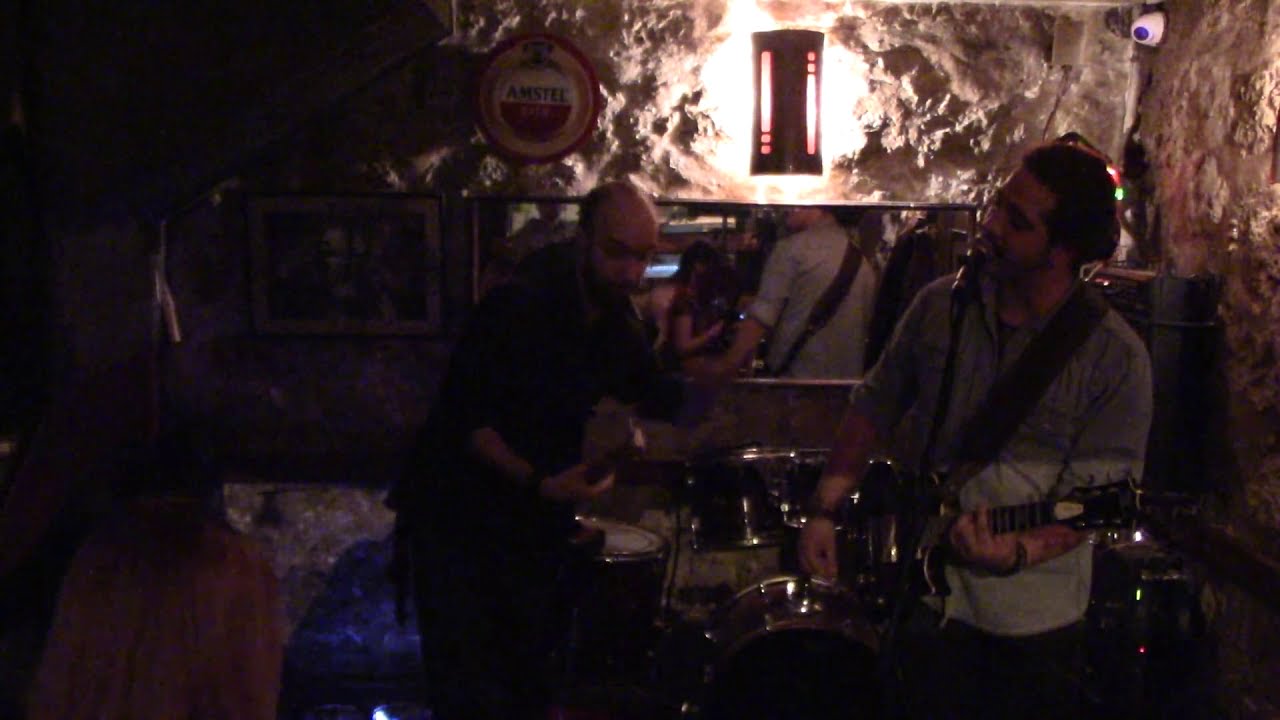The image depicts a dark, indoor setting that resembles a small bar or club. The walls have a rough, cave-like texture and are light brown in color. In the middle of the image, there is a band performing. To the right, a man with brown hair, wearing a blue button-down shirt, is playing a guitar and singing into a microphone. Slightly to the left, another man, dressed in dark clothing and balding, is playing a drum kit. The scene is illuminated by a single sconce light positioned above a horizontally long mirror on the wall behind them, which reflects the backs of both musicians. Hanging on the textured wall is an Amstel Light logo and some additional signs. In the upper right corner, a small security camera is visible. The band, centrally positioned, is the focal point of this atmospheric and artistically styled musical performance space.